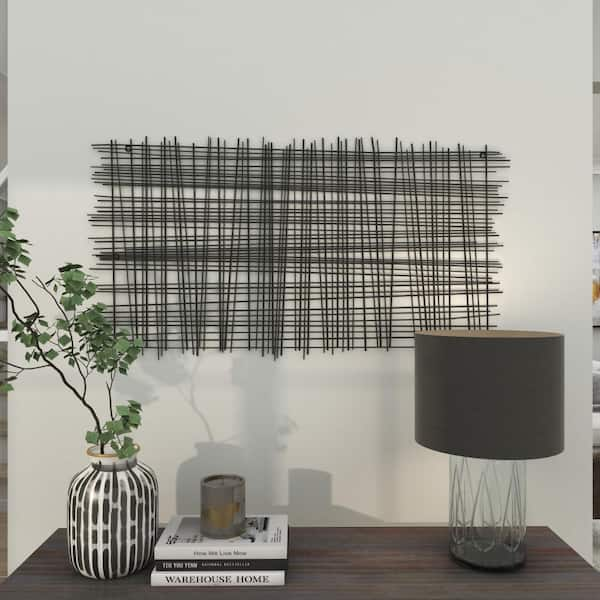This interior photograph captures a stylish and aesthetically pleasing tablescape set against a white wall. The focal point is a large piece of art on the wall, a reed mat with dark brown sticks woven in a grid of vertical and horizontal lines. Below the artwork is a wooden table adorned with several objects. On the right side sits a glass lamp with a short brown lampshade. Centrally, there is a stack of three books, with the only legible title being "Warehouse Home" at the bottom. Atop this stack rests a jarred candle. To the left of the books is a striped vase, from which branches with green leaves emerge and lean gently to the left. The overall scene exudes a minimalist yet inviting vibe, suitable for both home and office environments, and is reminiscent of images often showcased on social media platforms like Instagram.